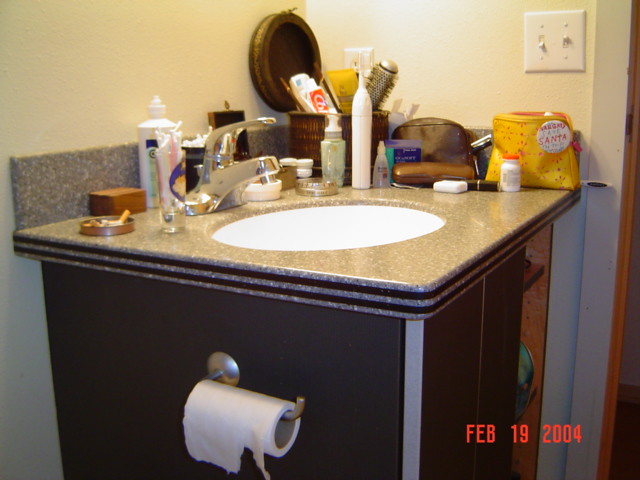The image depicts a cluttered bathroom sink area with numerous items scattered across a granite countertop that features distinctive brown stripes matching the base. The countertop, which has rounded edges, holds an ashtray overflowing with cigarette butts, indicating the space is not well-maintained. Despite the mess, the countertop itself is an elegant piece with alternating strips of granite and base color.

A toilet paper dispenser is attached to the side of the sink, confirming its location in a bathroom. However, the absence of a mirror above the sink is unusual. A light switch is visible on the wall, and the counter is crowded with personal items including a makeup bag adorned with a button that reads "Santa" and a small bottle of Tylenol in front of it. Another black makeup bag is present, with a probable eyeglass case and a container of dental floss in front.

Additional items on the counter include a bottle of eye drops, an electric toothbrush standing upright, a Lancome face cream pump, a container of cotton swabs, and what appears to be contact lens solution alongside contact lens cases. The cabinet below the countertop is partly open, revealing a green object inside. The overall scene suggests a lack of counter space leading to a messy arrangement of everyday essentials.